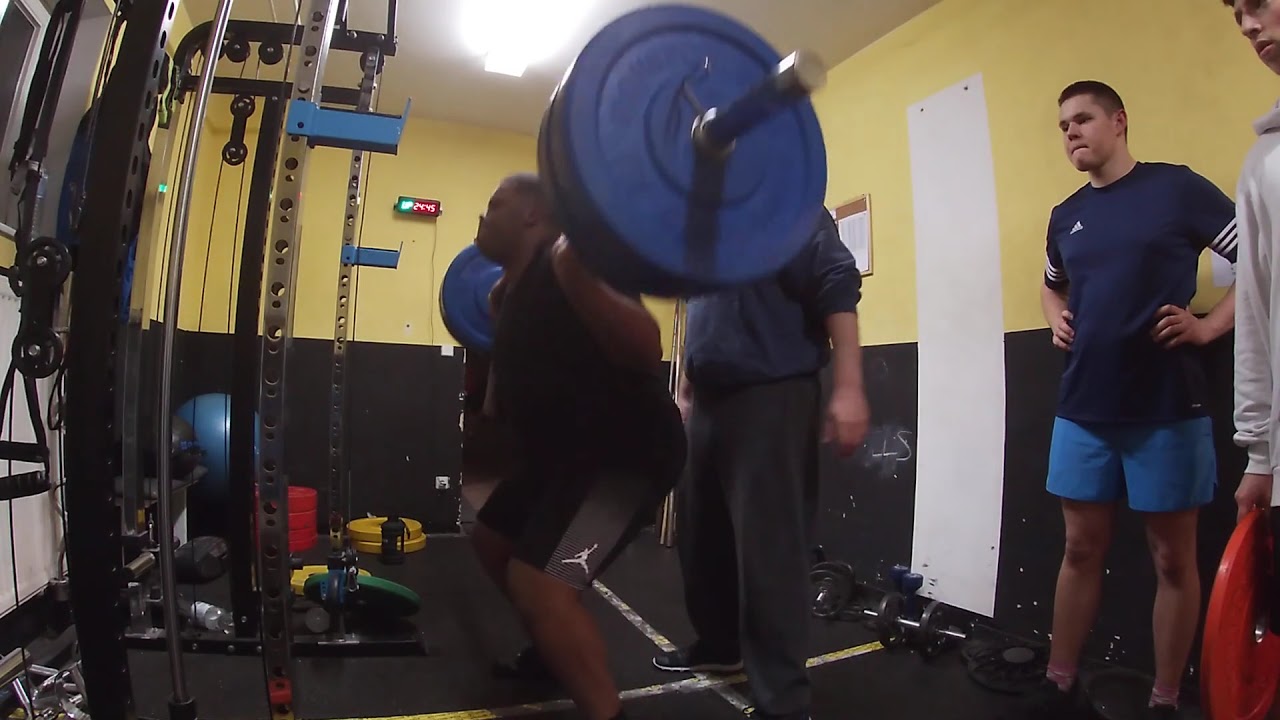In the image, a black man, dressed in a black tank top and black shorts, is captured in the middle of a weightlifting squat. He has a barbell with large, round weight discs positioned behind his shoulders, and he's bent slightly forward at the knees and back, with his head leaning backward. Behind him stands a man with a bearded gut, identifiable by his dark blue shirt and long, dark gray pants, possibly serving as a spotter. To the right of the lifter is another man with a grimacing expression, wearing a navy blue Adidas shirt with white stripes on the sleeves and light blue shorts, grabbing the sides of his waist. There is also a fourth individual in a grayish jacket holding a red weight disc, observing the lifter. The gym setting is evident from the presence of various weightlifting machines, a Powerball in the background, and the distinctive yellow upper and black lower walls, as well as the black flooring.